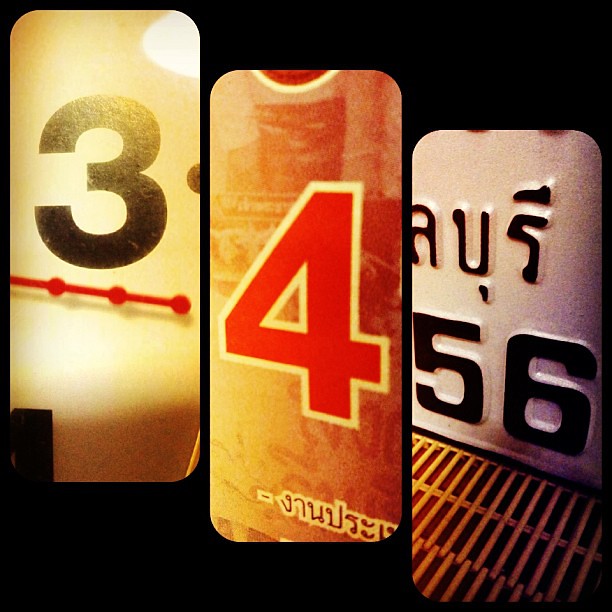The image is a triptych collage with a black background, featuring three tall, vertical rectangles with rounded corners that descend diagonally from the upper left to the lower right. Each rectangle showcases a number in distinct styles:
- The leftmost rectangle has a tan background with a large, bold black number "3". Below the number, there is a red line with three spaced-out red dots.
- The center rectangle features a red number "4" with a yellow outline on a light brown or reddish background and includes some writing in a foreign script, possibly Thai or Arabic.
- The rightmost rectangle displays the numbers "5" and "6" in bold black on a white background. Beneath the numbers, there’s a golden metal grate-like element and additional foreign text.

Each number appears as if displayed on distinct signage or license plates, contributing to an eclectic visual flow from the top left to the bottom right of the image.